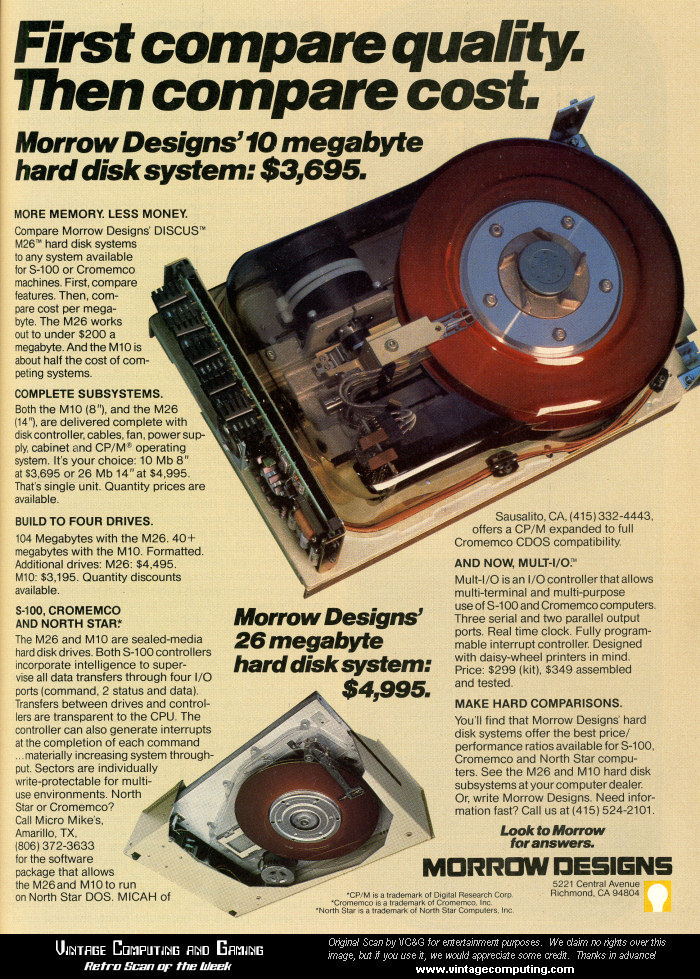This advertisement, seen against a bright yellow background, promotes Morrow Designs' hard disk systems with a compelling headline: "First compare quality, then compare cost." Featured prominently is the 10-megabyte hard disk system, priced at $3,695. The ad also highlights another product, the Morrow Designs 26 megabyte hard disk system, available for $4,995. 

The layout includes a large picture of a hard drive accompanied by detailed text sections that describe the product's features and benefits. Additionally, a smaller image of the hard drives is presented below. The text emphasizes the key selling points: "More memory, less money," and encourages consumers to compare Morrow Designs' Diskus M26 hard drive systems with any competing system available for S100 or Cromemco machines. 

Highlighted features include complete subsystems built for configurations with up to four drives, compatible with S100, Chromemco, and North Star machines. The advertisement targets vintage computing enthusiasts and is associated with a website, www.thevintagecomputing.com, which is mentioned at the bottom, alongside the tagline "vintage computing and gaming, retroscan."